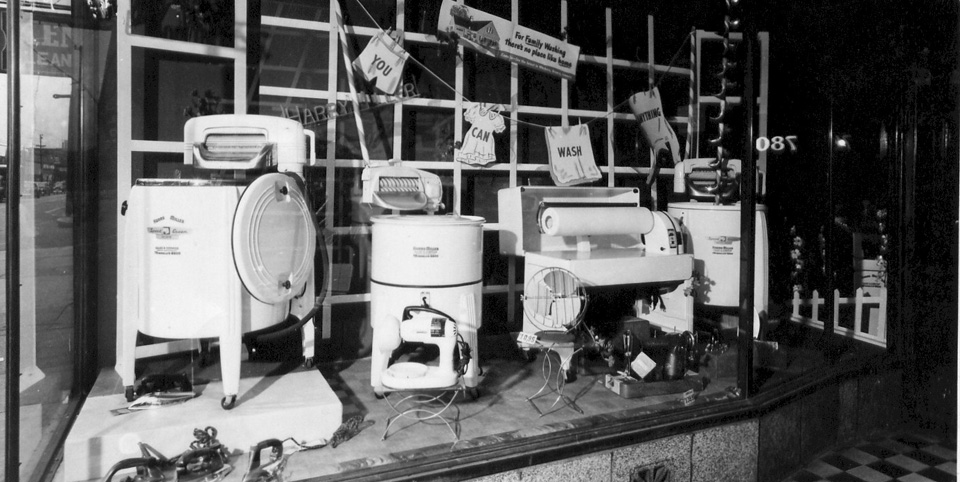This vintage black and white photograph captures the front display of an antique appliance store, showcasing an array of old-fashioned household items. Central to the display are several early-model washing machines, equipped with wringers mounted on arms above them, reminiscent of large, mechanical stand mixers. The scene is framed by a deep bay window, with a reflection indicating the store's address as 780. Notably, the display includes a caged fan, plug-in irons, and a large rolling press, suggestive of industrial washing equipment.

The backdrop is adorned with a clever advertisement styled as a clothesline, where garments shaped signs spell out "You Can Wash Anything," each letter printed on items like a pair of shorts, a frilly dress, a towel, and a shirt. Additional small signs in the background read uplifting messages such as "For Family Working There's No Place Like Home."

The sidewalk outside the store features a black and white checkerboard tile pattern, emphasizing the historical charm of the setting. Though the glass is clear, allowing a view of the appliances and the decorated background, the interior of the store itself remains obscured. The absence of people heightens the nostalgic atmosphere, focusing attention on the bygone era's technological marvels.